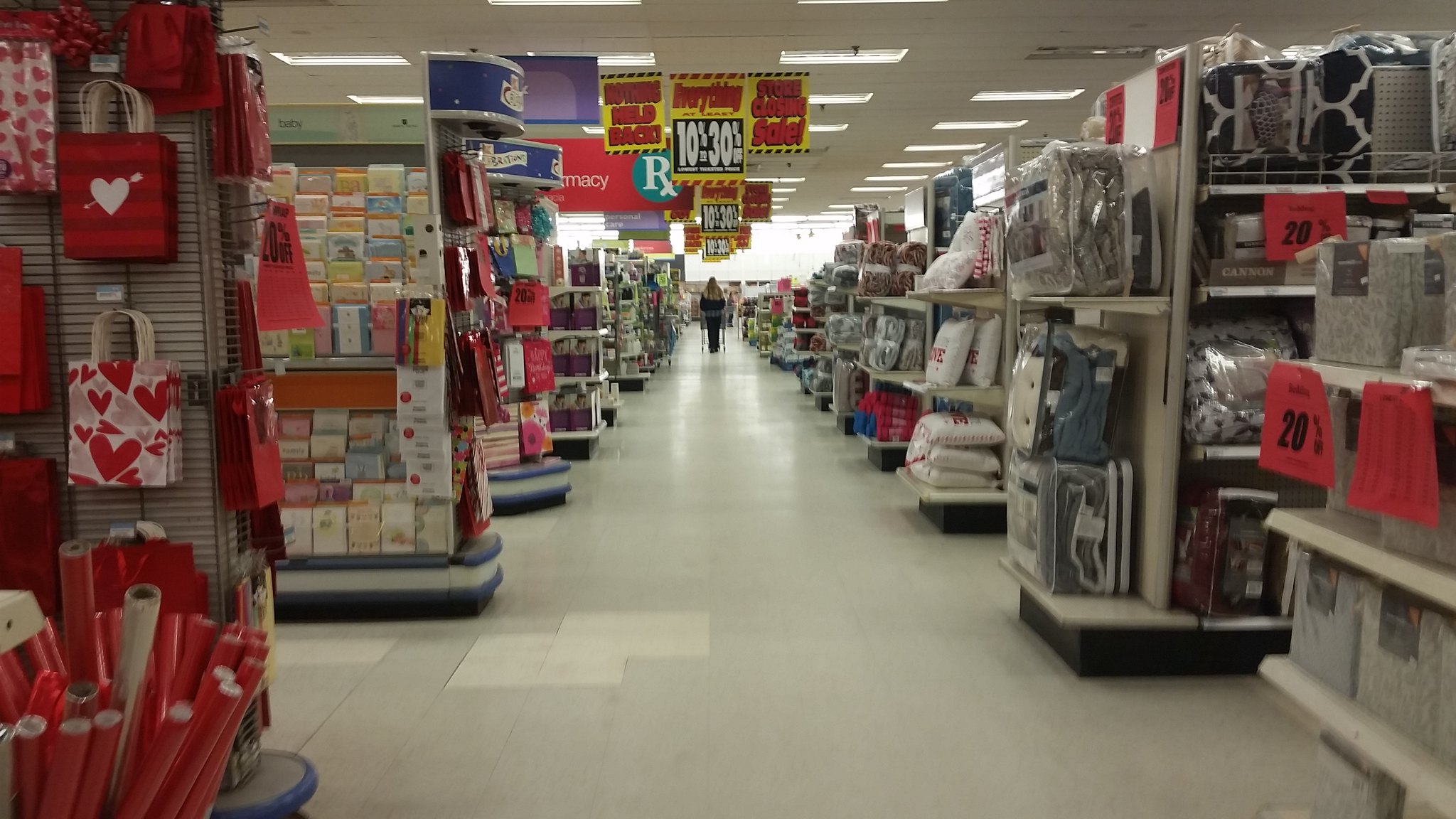The photograph captures the bustling interior of a department store, likely taken around Valentine's Day. Central to the image is a wide, open aisle bordered by a variety of product displays. On the left side, there’s a prominent Valentine's Day section adorned with vibrant red wrapping paper and gift bags, followed by a section of greeting cards. Further down, though less discernible due to the distance, are additional product displays.

To the right of the aisle, the displays primarily feature housewares. Closest to the camera are neatly arranged blankets or bedspreads, followed by pillows, and further back, more blankets and assorted houseware items.

A woman with long blonde hair, dressed in black, can be seen pushing a shopping cart in the distance down the aisle. Overhead, the ceiling is fitted with lighting panels, and various signs hang down, advertising sale prices and discounts throughout the store.